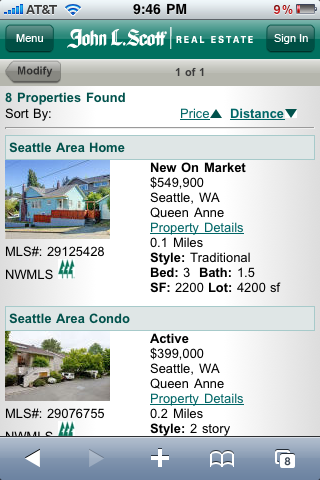The image is a screenshot taken on a mobile device, either a phone or a tablet. At the top of the screen, the status bar shows the AT&T carrier signal strength, the current time, and the battery life. The main content is a webpage from the John L Scott Real Estate website, featuring a green label with white text displaying the company's name.

Below the label, there is a search result page showing various houses for sale. The interface includes clickable options such as filtering by price or distance, indicated by arrows beside each option. The top of the search results section states "8 properties found," although only two listings are visible in this screenshot. Each listing provides a detailed description of the homes, including the price and the type of property.

At the bottom of the screen, there is a gray navigation bar typical of mobile devices, featuring buttons for going back, viewing open tabs, and accessing other device functions.